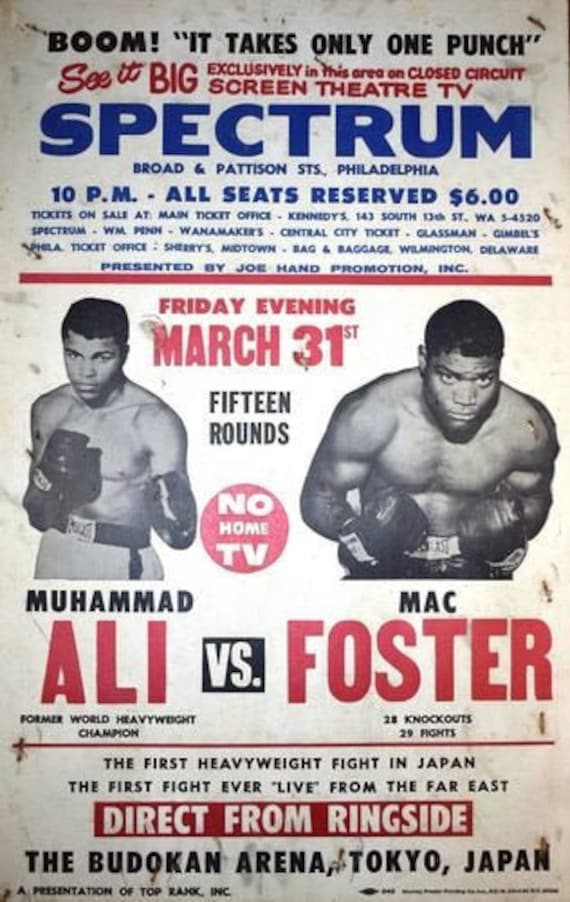This vintage poster advertises a historic boxing match between Muhammad Ali and Mac Foster. In the center, the poster prominently features black-and-white photos of Muhammad Ali on the left and Mac Foster on the right, with their names labeled beneath their images. Above these photos, bold black text proclaims, "Boom, it takes only one punch." Highlighted in red, the text urges viewers to, "See it big exclusively in this area on closed-circuit screen theater TV," while in blue, the location is specified as "Spectrum, Broad and Pattison Streets, Philadelphia." Key details such as "Friday evening, March 31st," "15 rounds," and "No home TV," are also included in this section. The event time is noted as "10 p.m.," with "all seats reserved" for "$6." At the bottom, the poster heralds the global significance of the match, stating it is "the first heavyweight fight in Japan" and "the first fight ever live from the Far East, direct from ringside, the Budokan Arena, Tokyo, Japan."